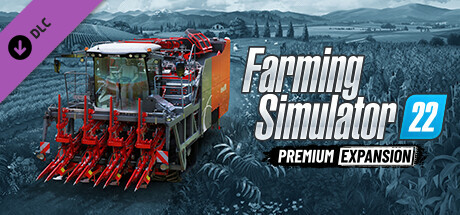The image is an advertisement for "Farming Simulator 22 Premium Expansion." Dominating the foreground is a large piece of farm equipment characterized by bright red cutters at the front, an orange seed box at the back, green panels, and a white roof. Inside the cab, two people are visible, one driving and another sitting next to them. The backdrop is an expansive farm field rendered in muted tones of grayish-green, with crops, likely corn, visible to the left of the image. In the distance, hills, a semi-circular building, and mountains are faintly outlined. A prominent feature includes a purple diagonal banner in the upper left corner with a down-pointing arrow and the text "DLC." On the right side of the ad, the game title "Farming Simulator 22" appears in bold white text, with "Premium Expansion" beneath it, and a green leaf graphic with the number "22" in the middle, surrounded by a blue box.